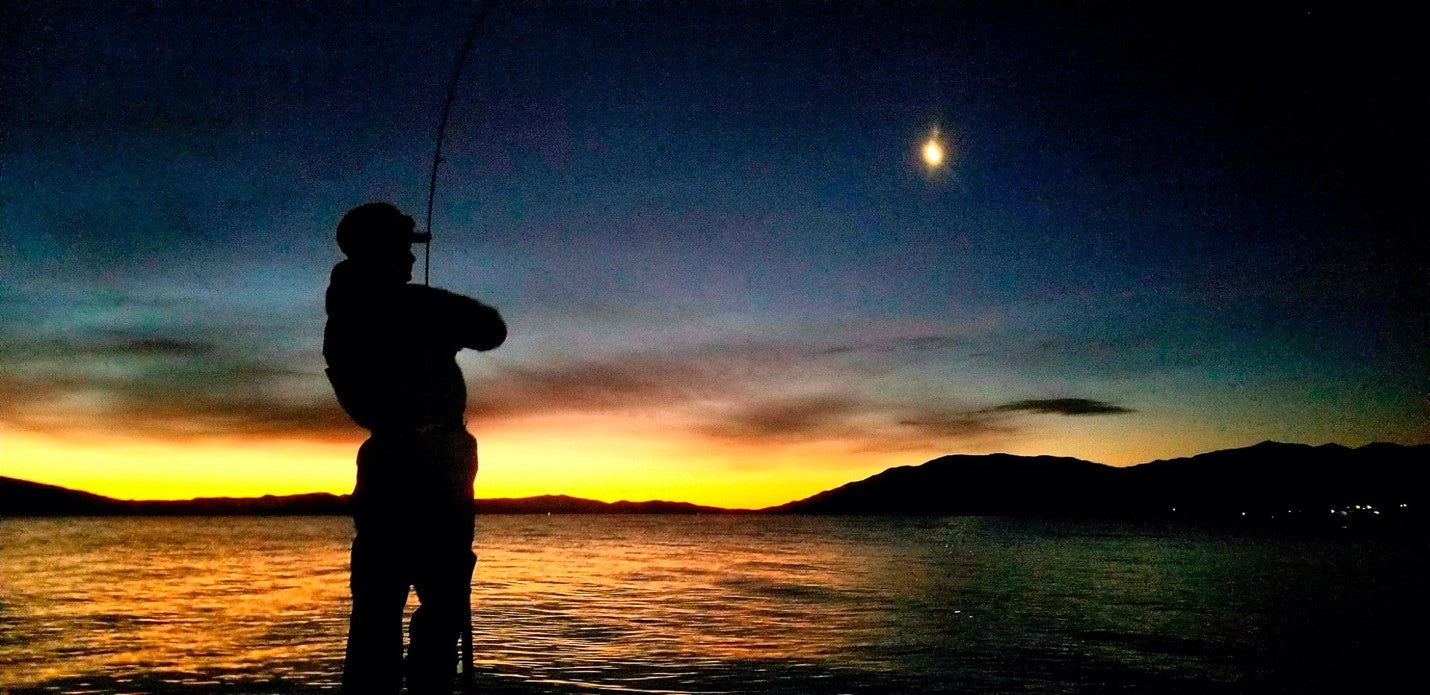In this image, a person, possibly an angler, stands on the shore of a large pond or lake during either sunset or sunrise. The figure, dressed in dark clothing and wearing a hat, has their back to the camera and is slightly turned to the right, holding a fishing pole that extends out of the frame above them. The foreground is dominated by the tranquil, shimmering water reflecting the varying hues of the sky. The lower part of the photo features a distant landmass stretching across the entire width, with an array of small town lights visible on the right-hand side. The sky is a rich tapestry of colors: starting with a deep, dark blue at the top corners, transitioning to soft whispering gray clouds, then a thin band of yellow near the horizon. Above the yellow band, a large, bright light—possibly the sun or moon—shines in the left-of-center top half of the image. The overall palette and serene composition suggest a peaceful, almost night-time scene, enhanced by the faint illumination of what may be emerging stars and reflections in the water.